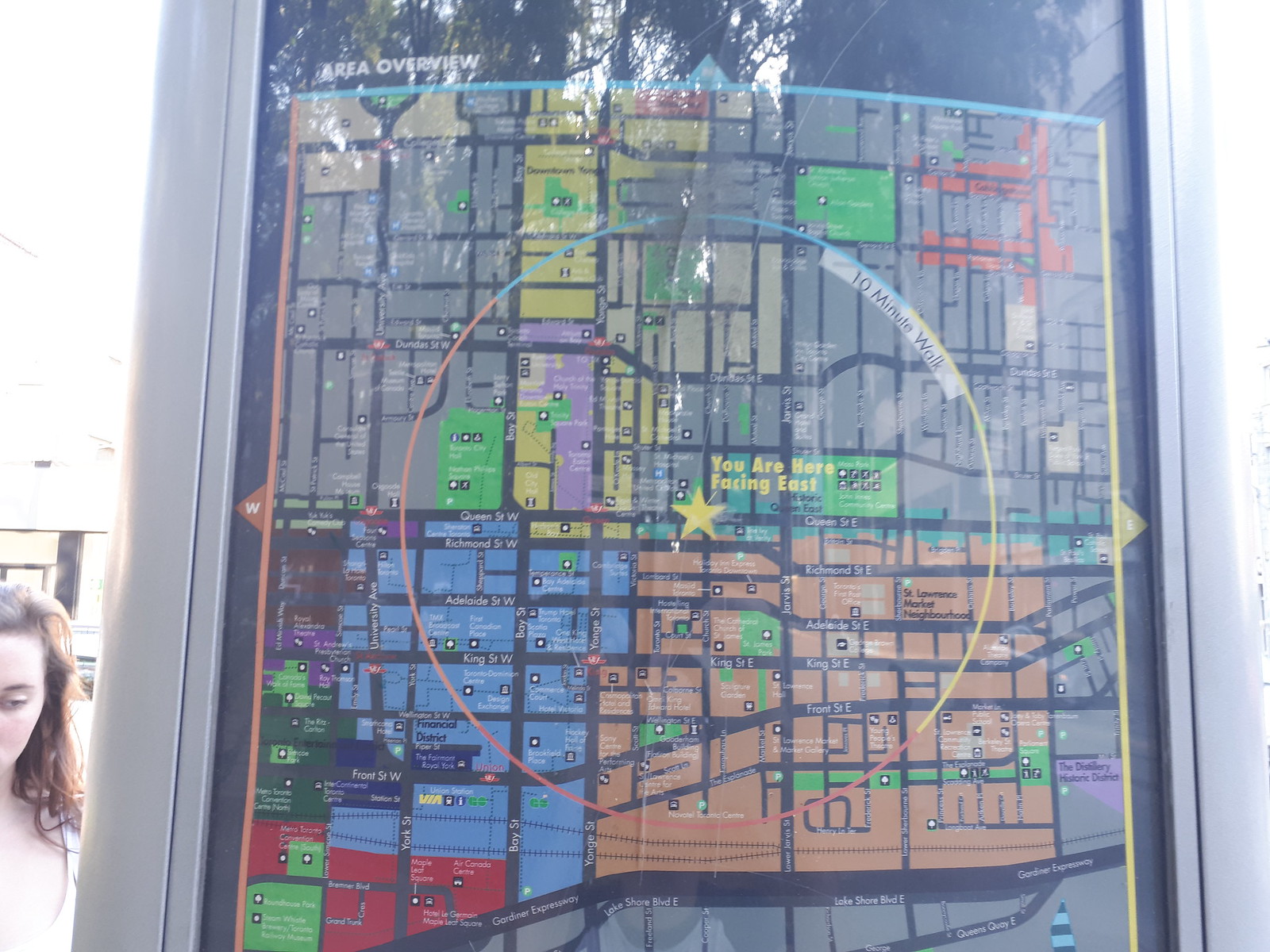The image depicts a detailed map display commonly found in large areas like malls. The map is held within a sleek, thin, silver frame with a glass panel. Dominating the right side of the image is the map, rich in colors - primarily orange, blue, green, yellow, gray, and black. Each color represents different sectors or functional zones, like streets or districts. Prominent street names on the map include Richmond Street West, Adelaide Street West, King Street West, Bay Street, Green Street, Front Street, and York Street.

At the top of the map is a title labeled "Area Overview." Various sections of the map are color-coded: a significant blue central area marked by a large circle labeled "10-minute walk," indicating areas that are roughly a 10-minute walk from the center. A star marks the "You Are Here" point, facing east. The map is bordered by different colored lines; blue at the top symbolizing north, yellow on the right for east, while south and west are likely represented but are partially cut off at the bottom of the image. The left border, signaling west, is marked in orange.

On the left side of the image, partially visible, is a woman with long, shoulder-length brown hair. Only the left side of her face is shown, with her left eye prominently visible. She appears to be studying the map, contributing to the image's context of wayfinding in a large area.